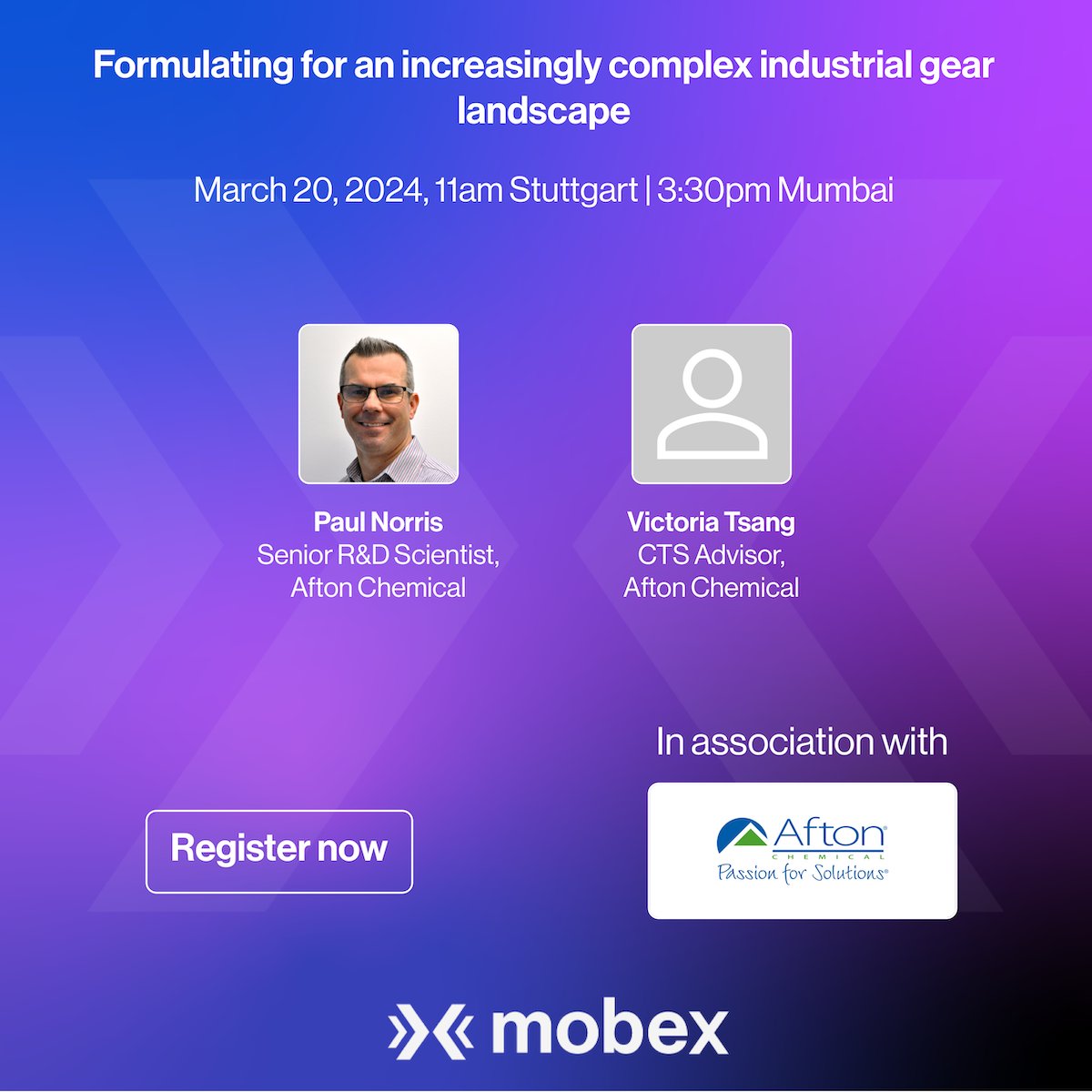This advertisement for Afton features a striking blue and purple background with arrows pointing towards each other from the sides, converging in the middle. At the top, in bold white lettering, it reads: "Formulating for an Increasingly Complex Industrial Landscape." Below this heading, the event details are provided: "March 20th, 2024, 11 a.m. Stuttgart / 3:30 p.m. Mumbai." Central to the poster is a smiling gentleman with very short hair and glasses, identified as Paul Norris, Senior R&D Scientist at Afton Chemical, wearing a collared shirt. Beside him, there's an outline of a head and shoulders representing Victoria Sang, CTS Advisor at Afton Chemical. In the bottom left corner, a clickable button in white lettering invites viewers to "Register Now." To its right, additional text in white letters states "Association with," positioned above a white box that reads "Afton Chemical." Finally, the poster credits Mobex in white text at the bottom.